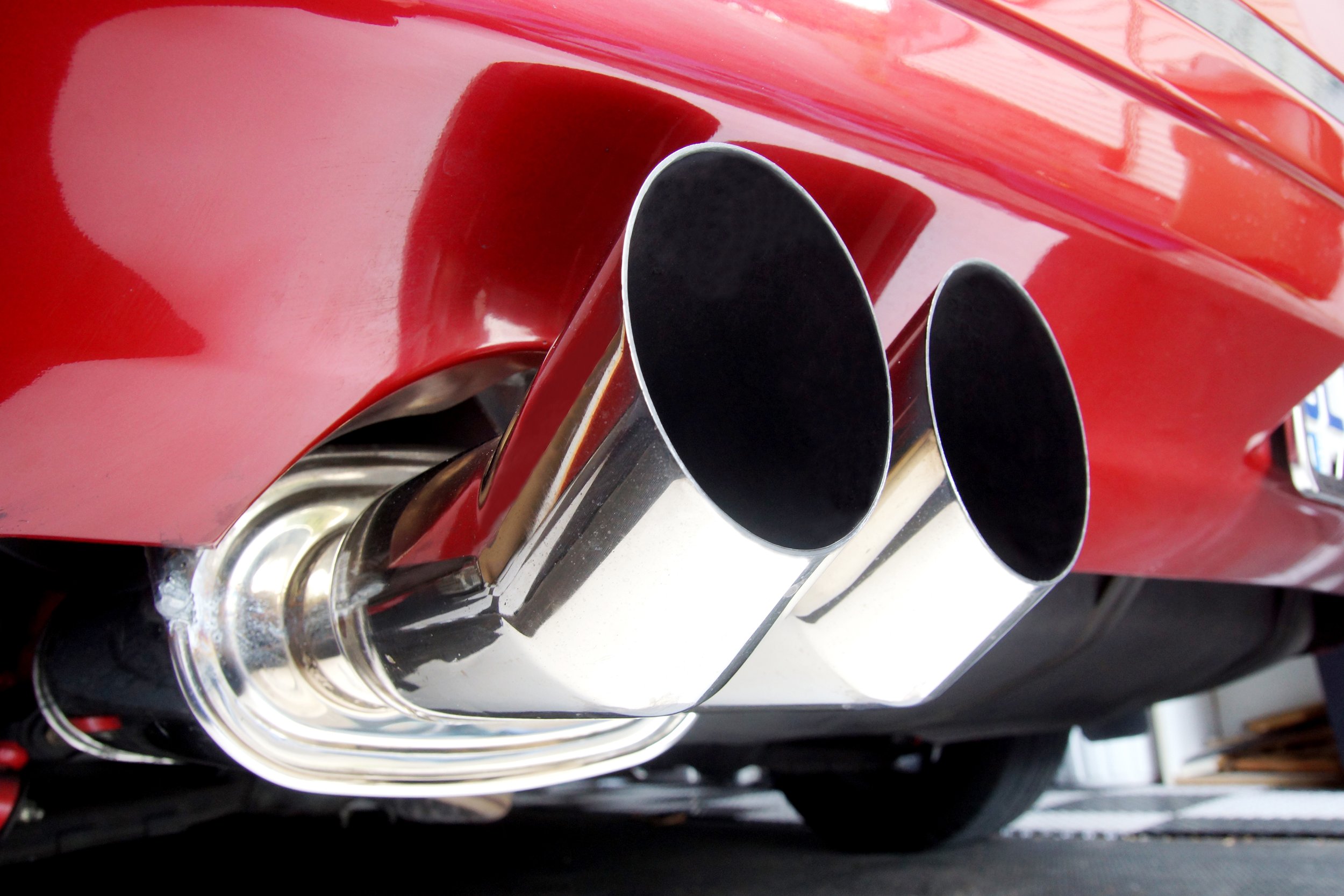The photograph depicts the underside and rear view of a shiny, bright red car parked on a paved, dark grey concrete street. Central to the image are the dual stainless steel exhaust pipes emerging from the bottom of the car, each curving upwards with a black circular interior. While the exhaust pipes dominate the left side, the right side features the edge of a license plate with visible letters "PL" on a name panel. The car's reflective surface gleams under the light, revealing its lighter red shade where the light hits. Additionally, a black air spoiler is visible beneath the exhaust pipes, hinting at the car's sporty design.